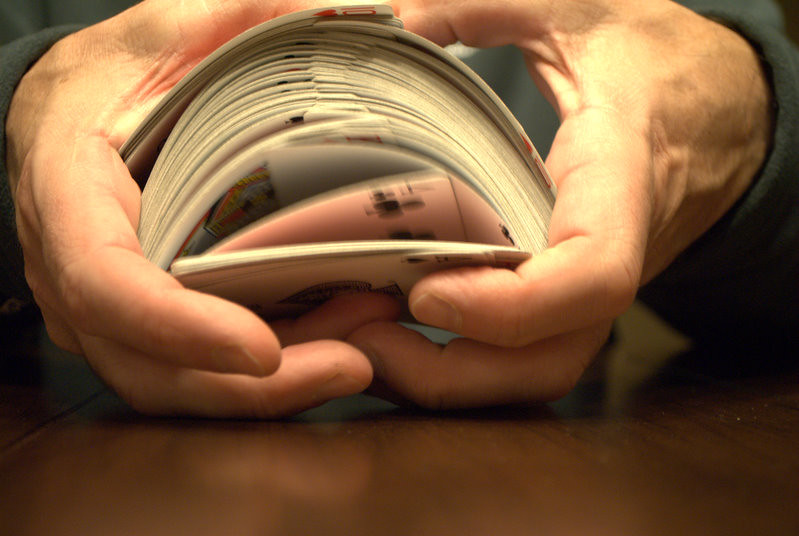In this high-quality image, we observe an individual in the midst of shuffling a deck of cards. The scene has a picturesque arrangement, with the camera strategically placed on a wooden table, capturing the action from a low, intimate angle. At the bottom of the frame, a portion of the wooden surface is visible, adding a rustic touch to the composition.

The shuffler’s hands, emerging from both the left and right sides of the image, are directed toward the camera. Between these hands, the cards form a wide and thick arch, suggesting the fluid motion typical of a professional shuffle. A small pile of already shuffled cards rests at the base of this arch. Some cards are in the process of interweaving, their edges beginning to align and merge, creating a slight blur that suggests motion. The faces of the cards in this movement are partially visible but indistinct due to the blur, adding a dynamic element to the photograph.